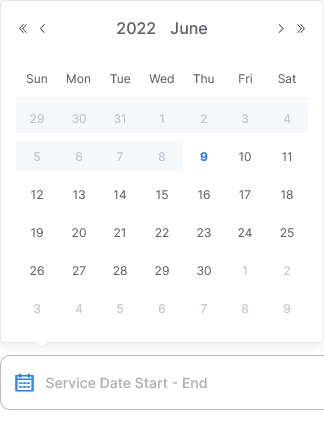The image is a screenshot of a digital calendar interface displaying the month of June 2022. On either side of the month and year at the top, there are navigation controls: two double arrows on the left side and a single arrow next to them, all pointing to the left, allowing users to navigate to previous months or years. Similarly, on the right side, there are two double arrows and a single arrow pointing to the right for navigating to future months or years.

In the middle of the interface, it clearly states "June 2022." The calendar grid below displays all the days of the month, with June 9th highlighted in blue, indicating it is the current date according to the screenshot. The number "9" is in blue, while all the other dates are in black or grey. June 9th falls on a Thursday in this calendar view.

At the bottom of the screenshot, there is a text box with the label "Service Date Start to End," accompanied by a small blue calendar icon on the left side of the text box.